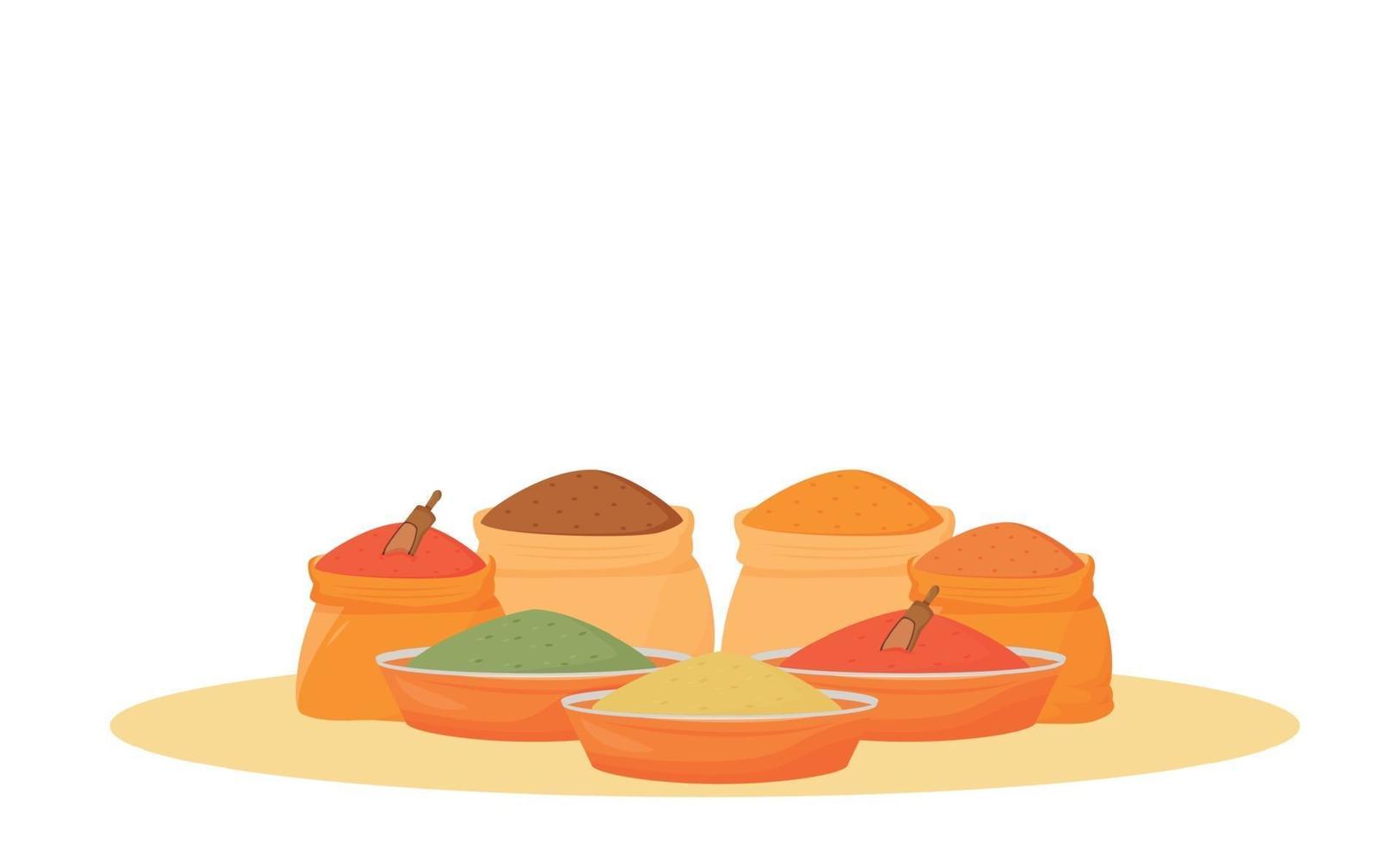This is a simplified, cartoon-like illustration depicting a display of various spices on a tan table. The arrangement features a yellow, circular plate as the base item. On the plate, in the background, there are four clay jars: two in dark orange and two in beige. Each jar is filled with different colored spices—red with a scoop, brown, yellow, and dark orange. Positioned in front of the jars are three orange bowls with white rims. The bowl on the left contains a green substance, the middle bowl holds a yellow substance, and the bowl on the right has a red substance with a small scoop sticking out of it. The background is completely white, highlighting the vivid colors and simple shapes of the items.